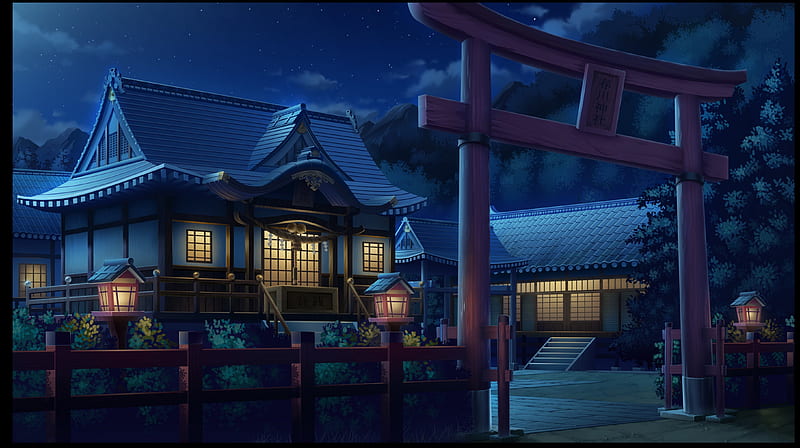The image depicts a night scene, illustrated in a style reminiscent of traditional Asian art, possibly from a location in China or Japan. Central to the scene is a large home showcasing quintessential East Asian architectural elements, such as roofs with curved bases and scalloped edges, and exterior walls with wood paneling. Surrounding the home is a fence, complete with ornate gateways marked by placards inscribed in Chinese. The fence posts are topped with lanterns, illuminating a pathway that leads to the property. The buildings within the scene are painted in rich shades of blue, accented by yellow lights and dark brown tones. Their windows and doors are framed with intricate grids, adding to the authenticity of the Asian aesthetic. In the background, tall pine trees and a glowing moon cast a serene ambiance over the landscape, further enhancing the multi-layered, mystical atmosphere. The image is horizontally rectangular with a black border, emphasizing the depth and complexity of the night scene.